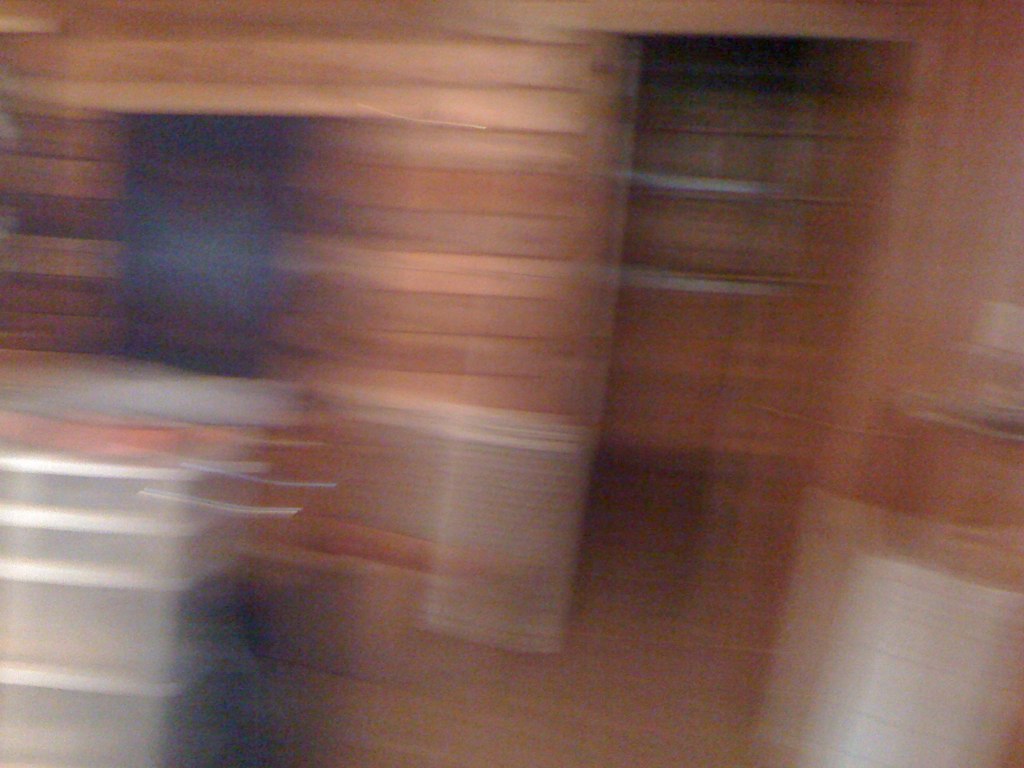This image, although very blurry and pixelated, appears to depict the interior of a room, likely a kitchen, in a house. The back wall seems to be made of wood paneling with various shades ranging from lighter wood, gray, to darker brown, interspersed with some silver markings. There is a countertop nearby, possibly silver or holding silver items such as pots and utensils. On the left side of the image, there seems to be an island or storage containers stacked with clear plastic and white lids. Additionally, the room features silver shelving and vents. In the top right section, a doorway can be discerned with two silver braces or brackets. On the left wall, a black sign or poster with red and white elements is visible. The overall graininess and blur of the photo make the details hard to distinguish, but these are the apparent features in the image.